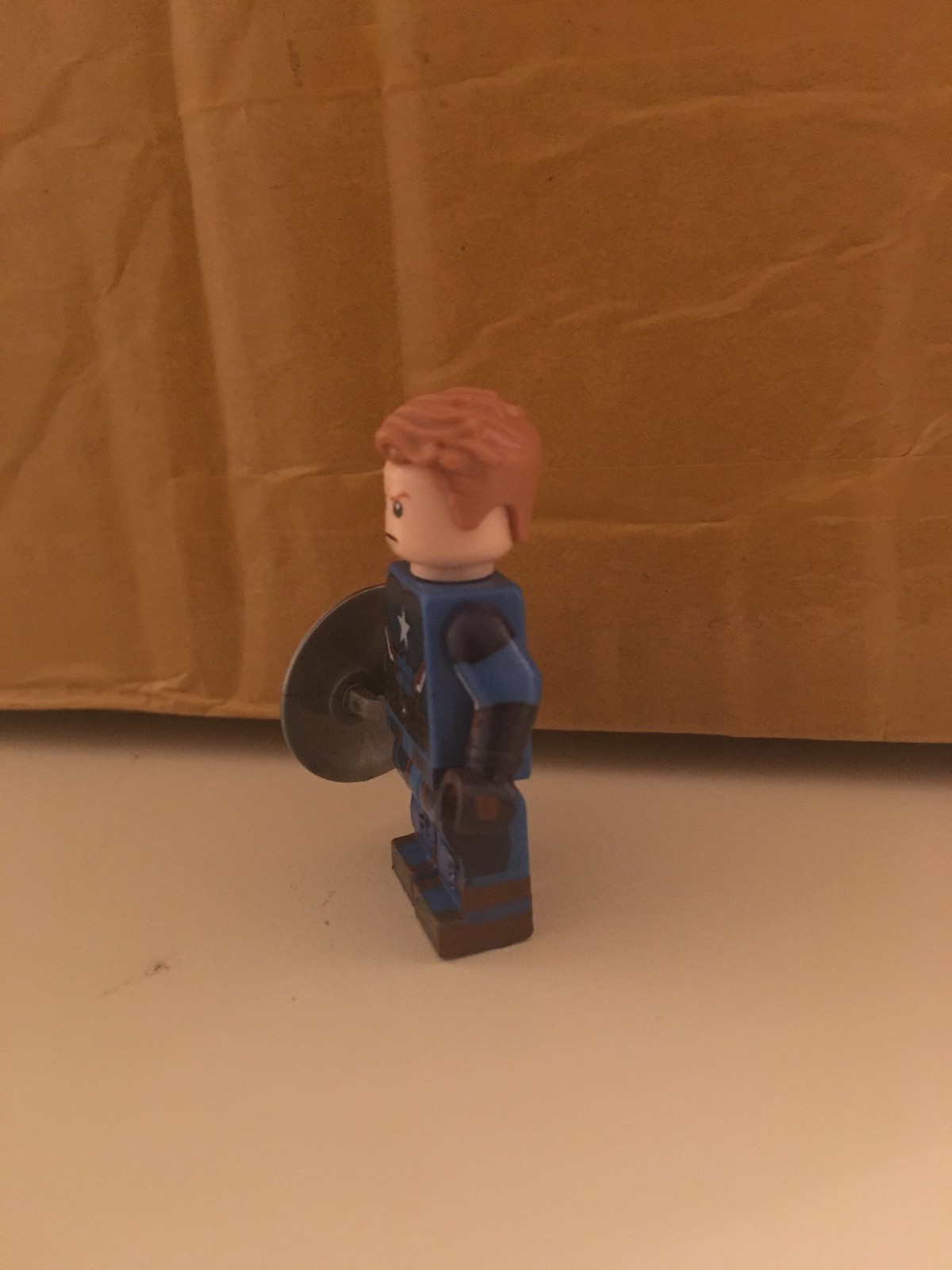This photo showcases a detailed scene featuring a small Lego figurine representing Captain America. The setting appears to be indoors, with the figurine positioned on a white or cream-colored table. The focal point is the Lego Captain America, characterized by his short brown hair, light skin, and determined expression with dark pupils. Dressed in a blue uniform adorned with a white star on his chest, he stands in a slightly angled stance, looking towards the left. Though his left hand is pointing slightly downward, his right hand holds a shield, which, despite not revealing its front, is identifiable by its distinct shape and position. The backdrop consists of a brown cardboard box, strategically placed to form a background. This box casting a shadow on the table adds depth to the scene, partially bent to create a hovering effect above the surface. The overall composition directs focus to the intricately detailed Lego Captain America, emphasizing both the craftsmanship of the figurine and the thoughtful arrangement of the setting.